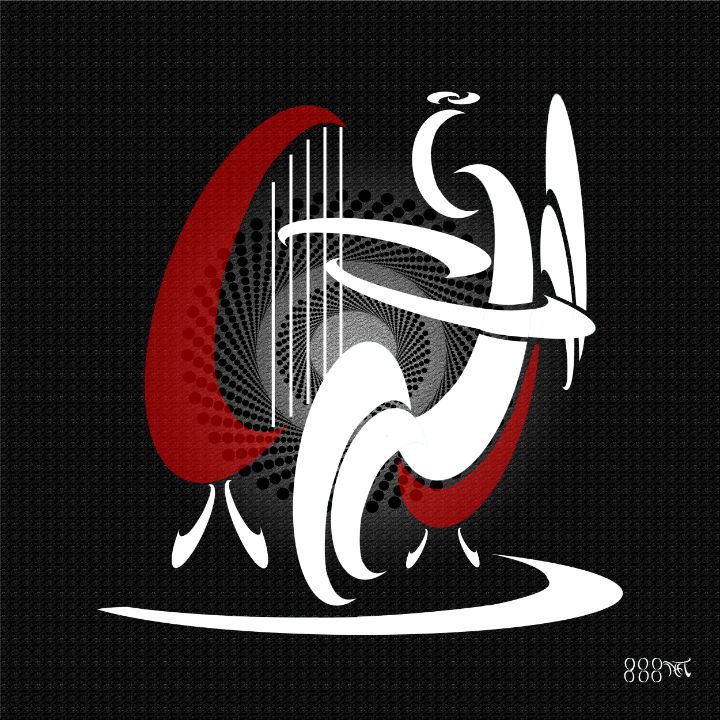This image portrays a visually intriguing abstract design against a textured black background dotted with tiny white or gray specs, lending it a tactile feel. Central to the composition are concentric rings of small black circles that fan outward, creating a layered, circular pattern. Dominating the left side of the image is a prominent red vertical swish, resembling a sideways 'C,' with two white slashes at its base, reminiscent of legs. To the right, an intricate assembly of white lines and curves coalesce, forming shapes suggestive of a bird-like figure with its tail down. These lines and swirls evoke the impression of quarter moons stacked and interwoven to craft a dynamic form. Beneath the central design lies a large reverse 'C' shape and a subtle maroon-colored curve that contributes to the sense of movement and flow. In the lower right-hand corner, the text "888NET" is cleverly integrated into the overall composition, enhancing the image's mystique and abstract nature.